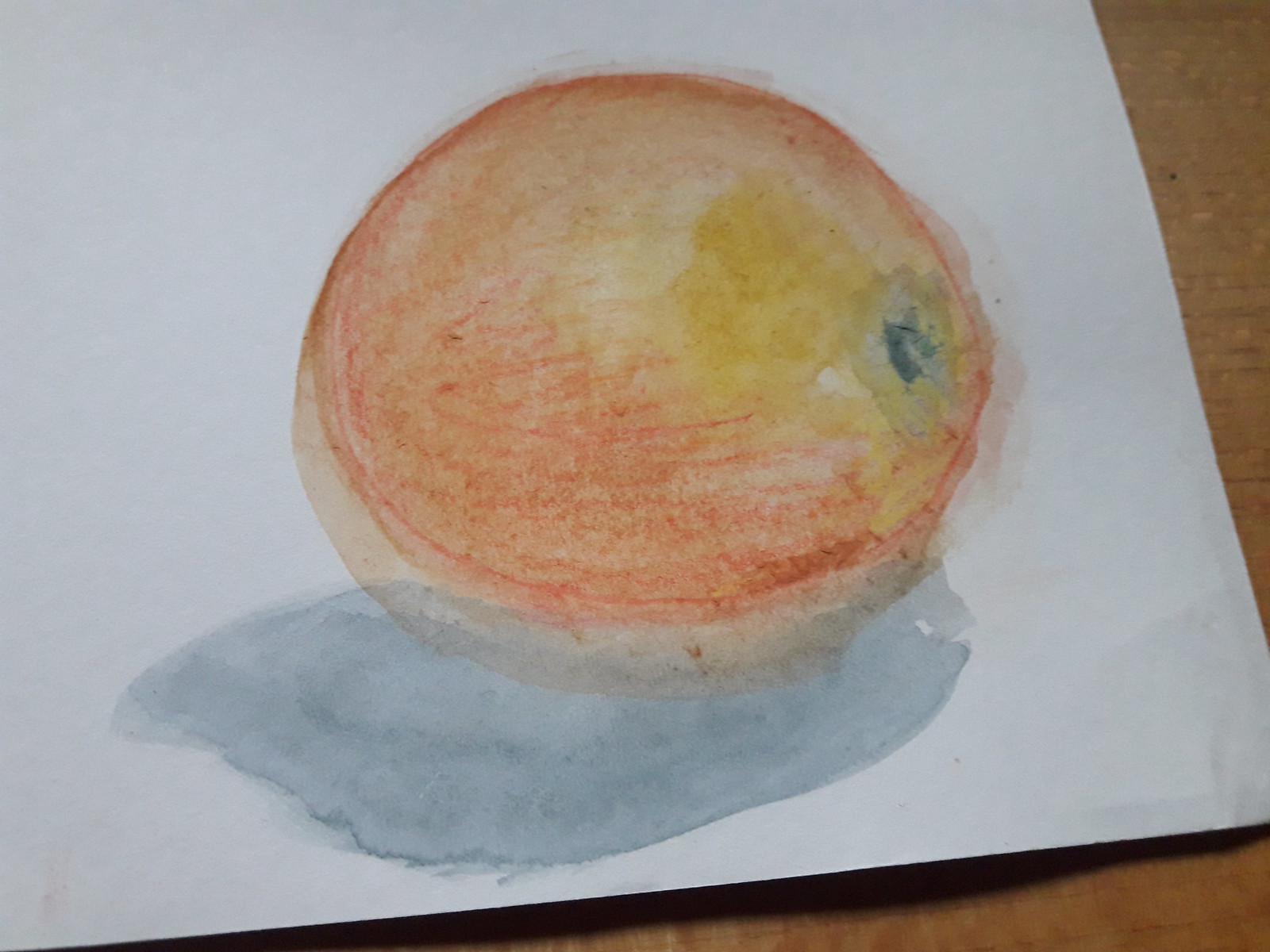The image depicts a watercolor painting positioned on a light brown wooden tabletop, with the paper covering most of the table surface. The white piece of paper features a circular, rounded object, potentially a fruit or a fish, illustrated with an orange to yellow gradient that transitions from dark orange on the outer edges to a creamy yellow center. In the upper right portion of the object, there is a distinct dark blue spot suggesting an eye, and below it lies a grayish light blue area that might represent a shadow or a water puddle. The artwork, though childlike in its simplicity, vividly showcases the contrasting colors and forms on the white canvas.